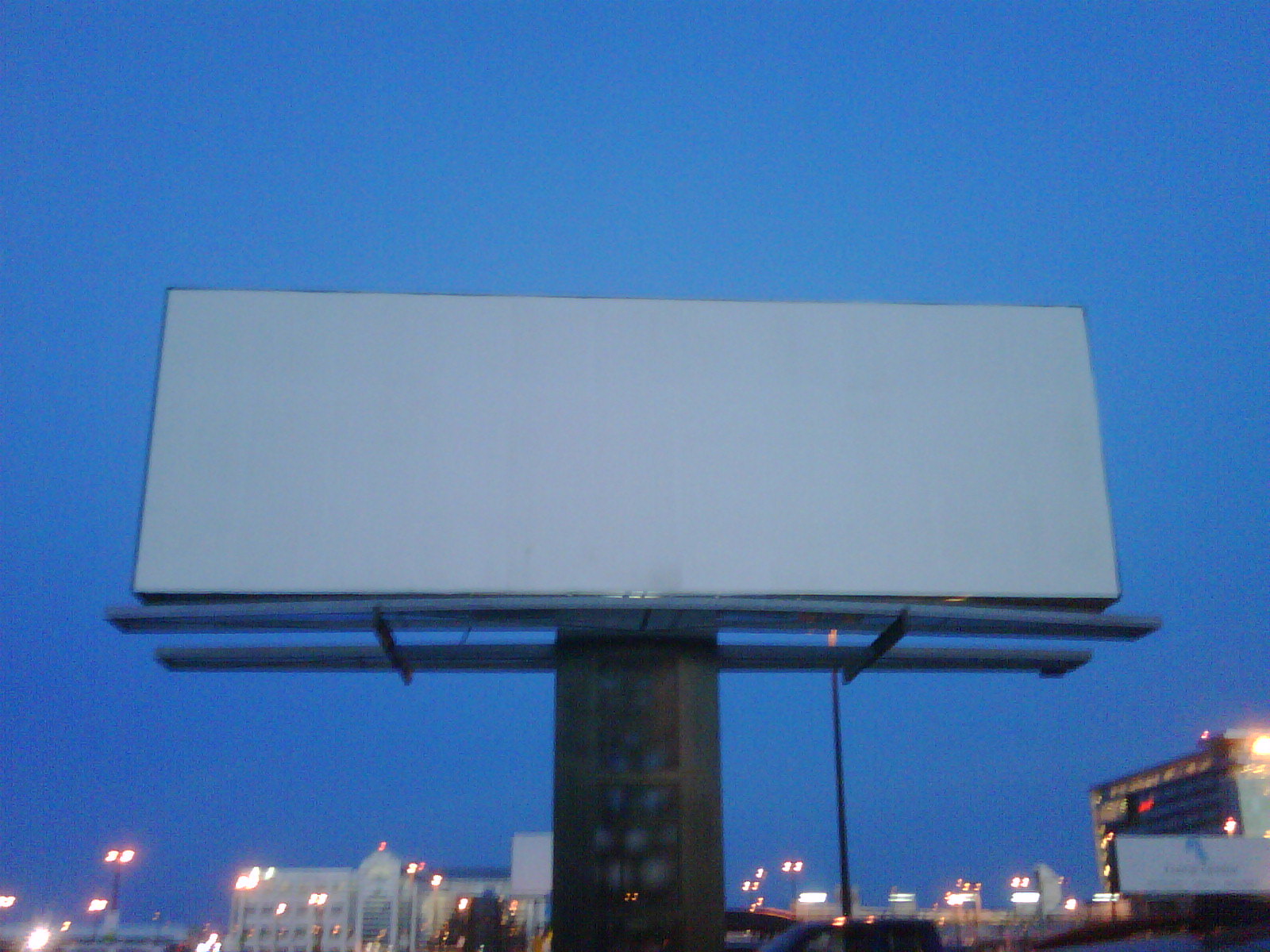In this image taken during the evening or at dusk, the sky exhibits a dark bluish hue, indicating the transition to nighttime. The cityscape in the background is illuminated, with lights shining from buildings and street lamps. The focal point of the photograph is a large, blank billboard elevated on a brownish-colored tower. The billboard itself is entirely gray or white, devoid of any advertisements or images. Supporting the billboard are two metal platforms, designed for workers to use while installing advertisements. To the right of the billboard, a tall building resembling a hospital stands prominently, while a white-colored, multi-story structure is visible in the background. Additionally, there is a white sign with a blue symbol and some black text on it positioned in the bottom right corner of the image, and in the bottom left corner, more buildings with yellow lights can be seen.